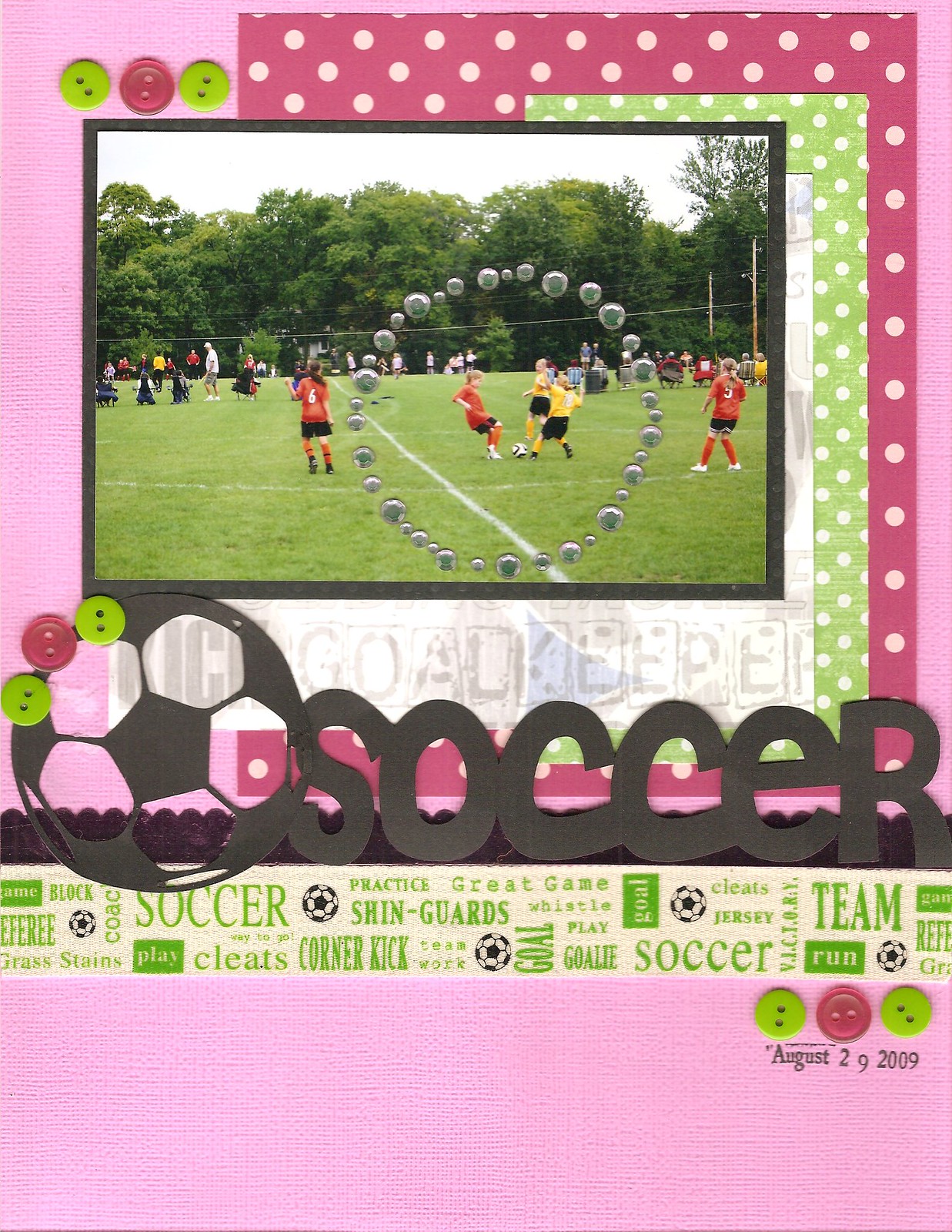This scrapbook page captures the vibrant memory of a young girl's soccer match, artfully displayed on pink construction paper layered with red and green polka dot accents. At the heart of the page, a daytime outdoor photograph showcases five young girls energetically contesting the soccer ball at the center of the pitch. Two girls don red and black outfits while their counterparts wear yellow and black. The action scene is adorned with sparkling bedazzled jewels, drawing attention to the spirited moment. Prominently featured below the photograph is the word “Soccer" cut out from black construction paper, paired with a black soccer ball illustration. Enhancing the collage are shirt buttons—two green and one red—strategically placed at the top left and bottom right corners. The date, August 29, 2009, is meticulously noted beneath the bottom right button, anchoring this cherished memory in time. The collage, with its animated elements and thoughtfully selected decorations, evokes the thrill and camaraderie of youth soccer.